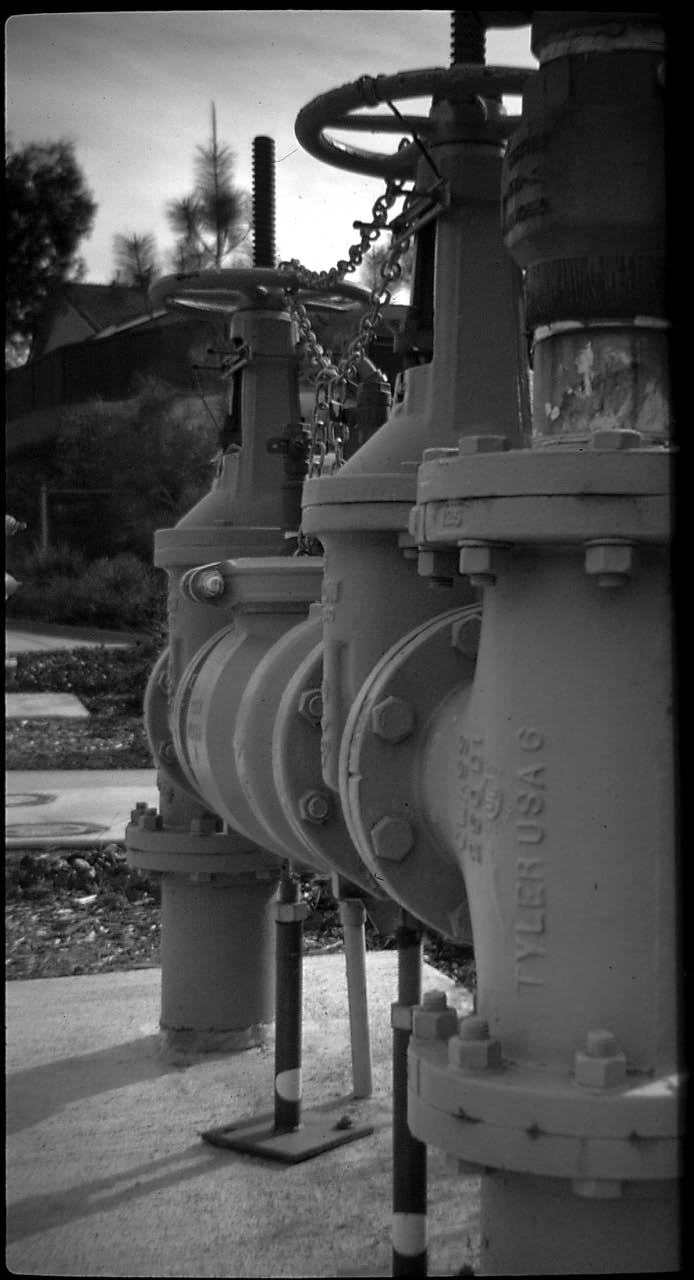This black and white photograph captures a detailed, up-close view of a series of large cast iron water shut-off valves positioned on a cement pad made of square slabs. The foreground is dominated by these interconnected valves, featuring embossed lettering "Tyler, USA" and equipped with wheel-style valve controls at the top. The valves are bolted together and secured with chains to prevent tampering, with smaller pipes branching off and leading into the ground. In the background, a house with a black roof is partially visible, flanked by various trees with dark gray leaves due to the monochromatic palette. The sky above is filled with light gray clouds, with patches that suggest the presence of sunlight diffusing through. The overall scene, with its rustic and industrial elements, emphasizes the outdoor setting, where shrubbery, bushes, patches of grass, and mulch contribute to the natural ambiance. Shadows cast by the water valves add depth and texture to this detailed depiction of historical infrastructure amidst its environment.